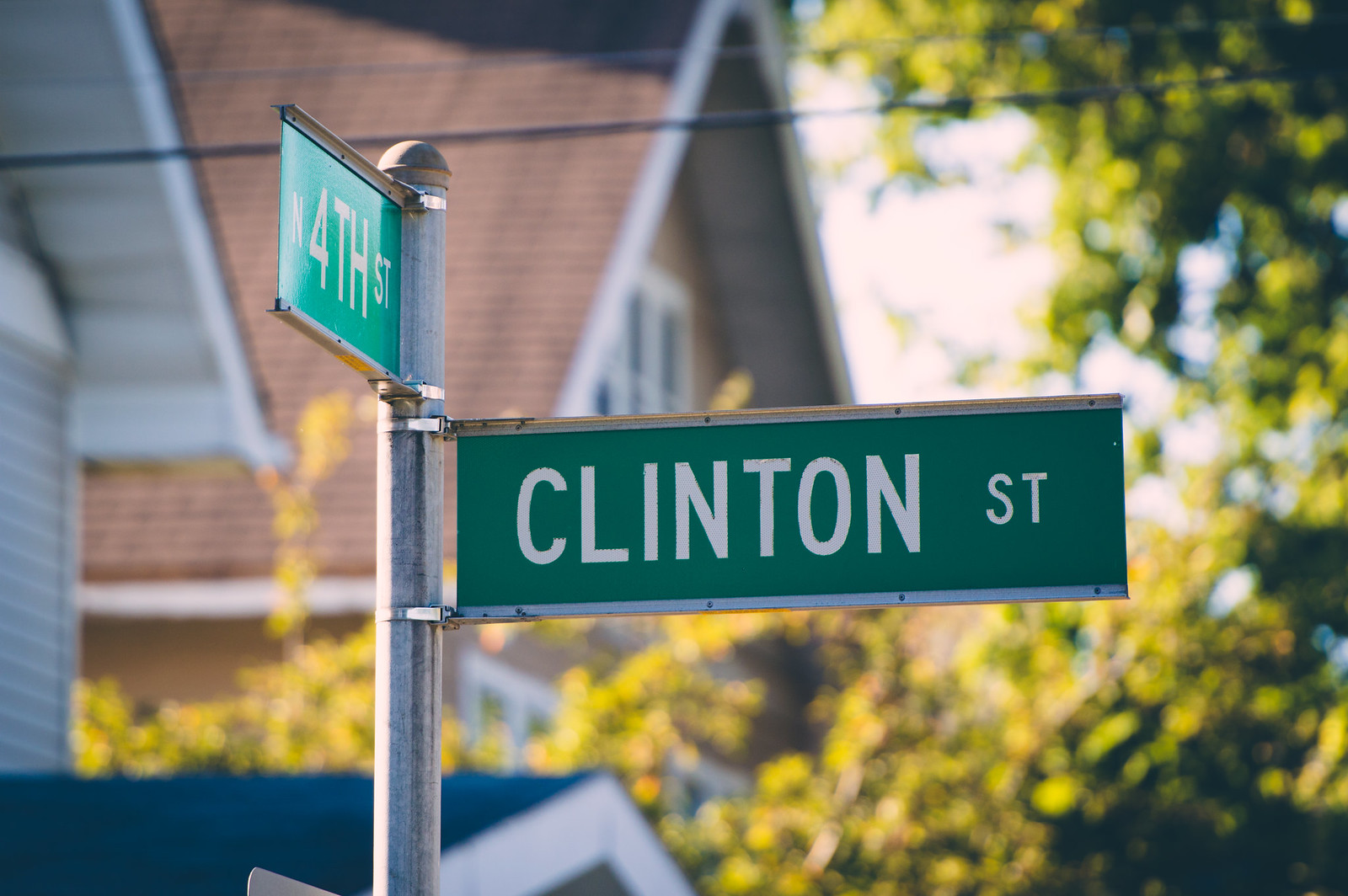The image displays two intersecting street signs mounted on a silver signpost. The signpost tilts slightly to the left, supporting a green rectangular sign extending to the right, labeled "Clinton Street" in bold white text. Above this, affixed perpendicularly, is another green sign pointing left, identifying "N 4th Street," also in white font. Overhead power lines crisscross the sky above the signs. To the right and along the bottom of the image, lush foliage from several trees is visible. Dominating the background is a brown house featuring a triangular roof with white trim and white-framed windows. Adjacent to it, to the left of the street signs, stands a blue house, providing a vivid contrast against the greenery and structures.